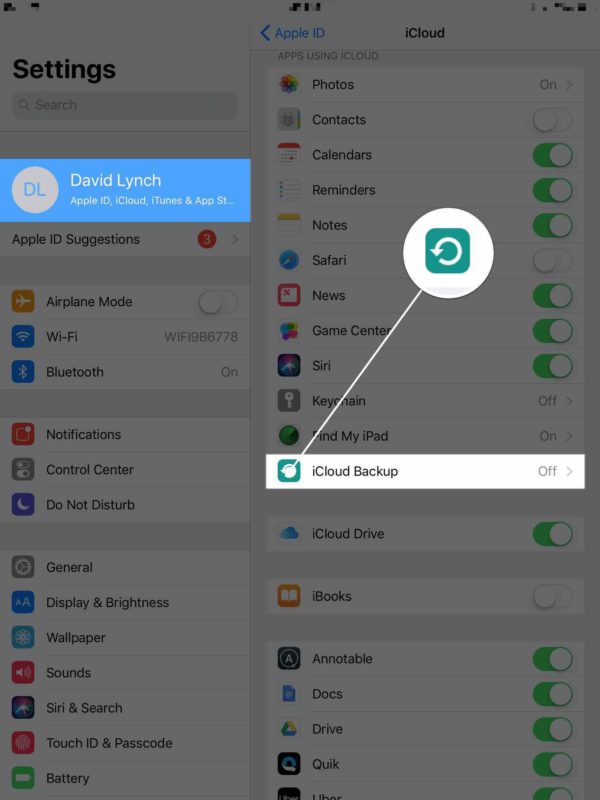In this image, the background is black and partially translucent, allowing a glimpse of settings beneath it. Dominating the central region is a blue rectangular box featuring a gray circle and a blue 'DL' insignia next to the text "David Lynch, Apple ID, iCloud, iTunes, and App Store." The interface displays various options like Apple ID suggestions, Airplane Mode, Wi-Fi, Bluetooth, Notifications, Control Center, Do Not Disturb, General, Display & Brightness, Wallpaper, Sounds, Siri & Search, Touch ID & Passcodes, and Battery.

On the right side, there's a top-header labeled 'Apple ID' accompanied by a left-pointing arrow and the word 'iCloud.' Below this are different settings categories such as Photos, Contacts, Calendars, Reminders, Notes, Safari, News, Game Center, Siri, Keychain, and Find My iPad. 

Additionally, there is a prominent white circle adjacent to a green box with a turn-around arrow. Below this, a large white line extends downwards to a smaller white box containing a green box with a white circle labeled 'iCloud Backup' with its status marked as 'Off' and a right-pointing arrow. Other elements visible include iCloud Drive, iBooks, Notable, Docs, Drive, and Quick.